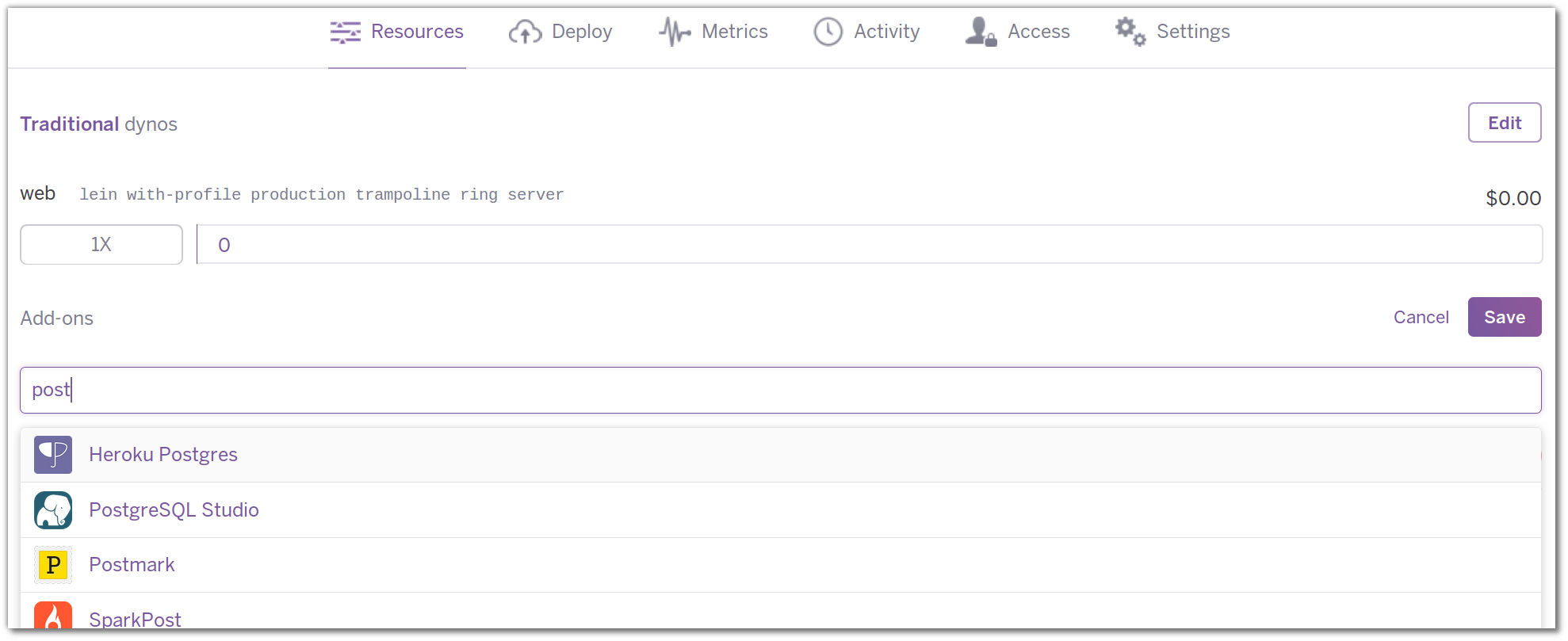Caption:
"A detailed view of a traditional Gynos web interface displaying the profile production settings and server options within the Heroku platform. The user interface includes various functional sections such as edit, cancel, save, post add-ons, and deploy configurations. PostgreSQL databases are managed through Heroku Postgres, with additional integrations for Studio Postmark and Spark Post resources. Metrics, activity logs, and access settings are prominently featured against a clean white background."